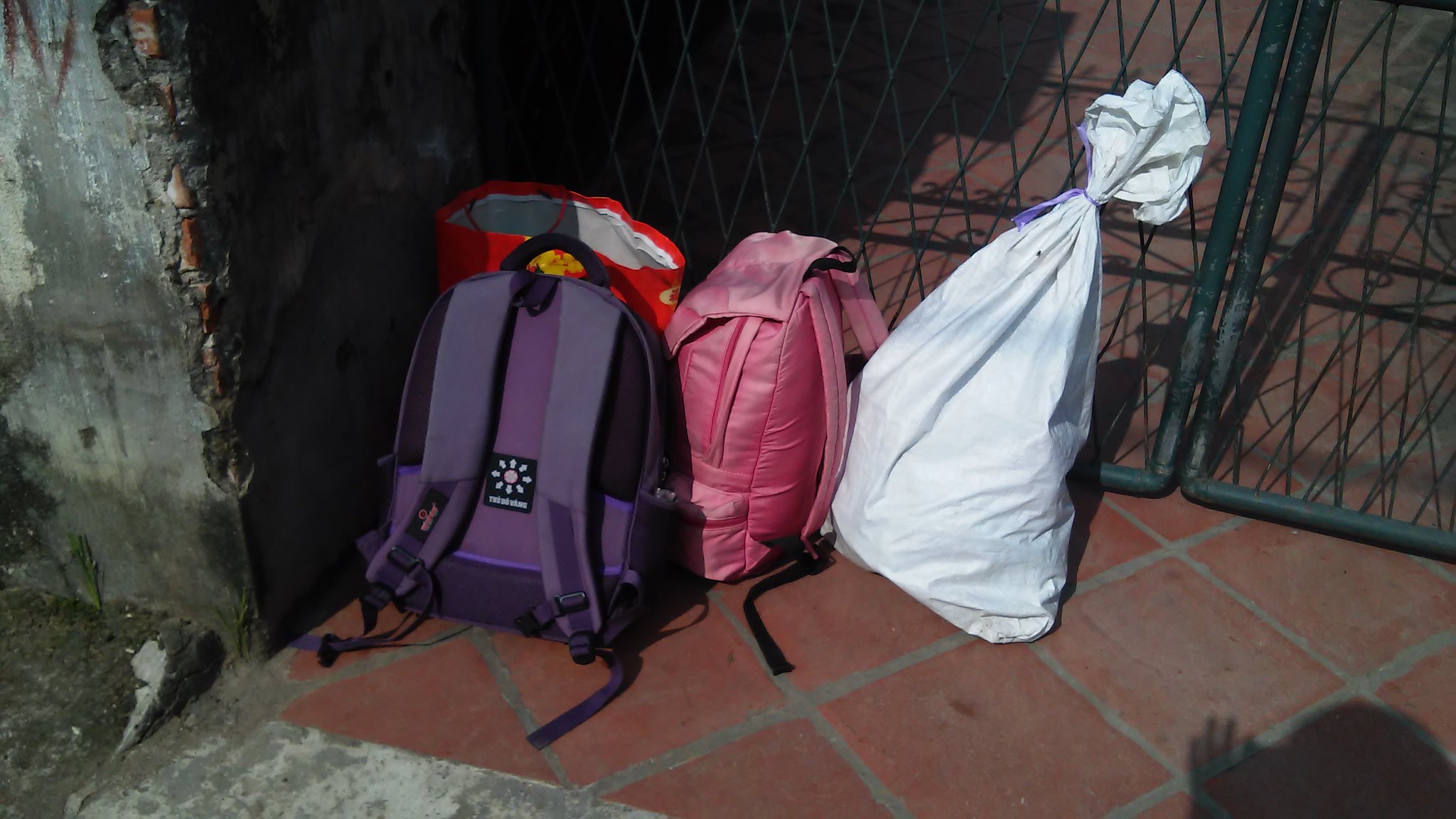This image, taken outdoors, depicts a collection of various bags placed on a red terracotta-tiled surface with visible gray grout lines. In the foreground, there is a purple backpack with its straps facing the viewer. Positioned behind it is a red canvas bag, which appears to have a white interior, possibly indicating it is insulated. To the right of the purple backpack is a pink rucksack, slightly tilted with its straps also visible. Further to the right is a white plastic bag, which is tied at the top with a purple string. The scene is set against a backdrop of a concrete wall on the left, which transitions into a black metal gate featuring a diamond-shaped mesh pattern. There are small patches of gravel and some evidence of plant growth near the concrete wall, adding texture to the environment. The shadow of the person taking the photo can be seen in the bottom right corner, suggesting the image was captured in natural light.